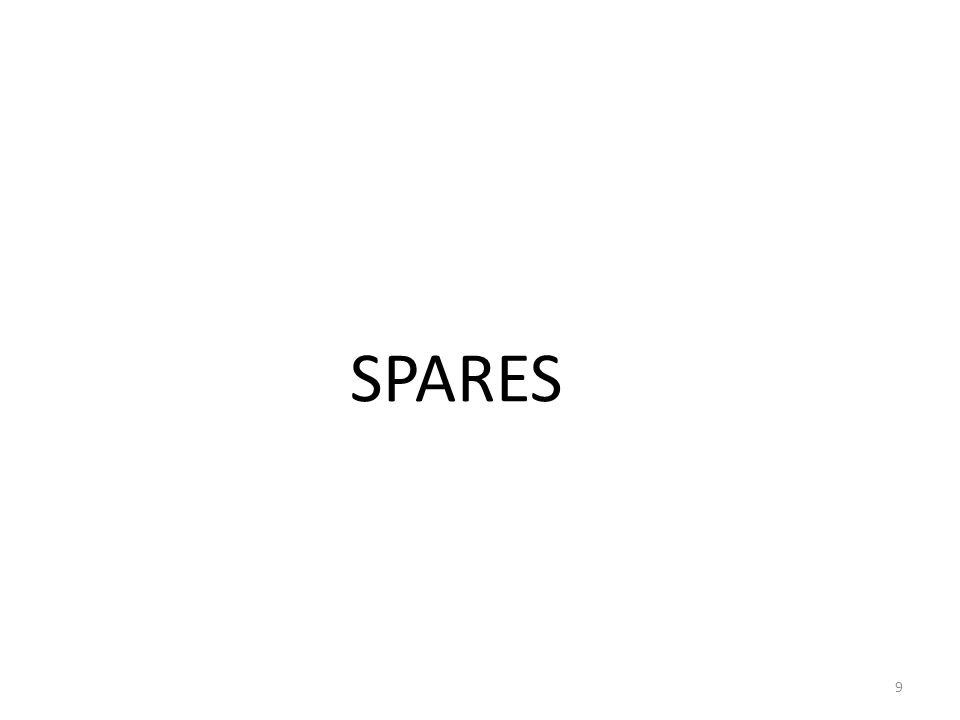The image features a minimalist design with a completely white background. In the left center of the image, there is a single word in all capital letters: "SPARES," rendered in a sans serif font that resembles Helvetica. The black text is relatively small compared to the overall space of the image but remains the dominant feature. In the bottom right corner, there is a tiny number 9 in a grayish color, significantly smaller than the main text. There are no other objects or colors present in the image.